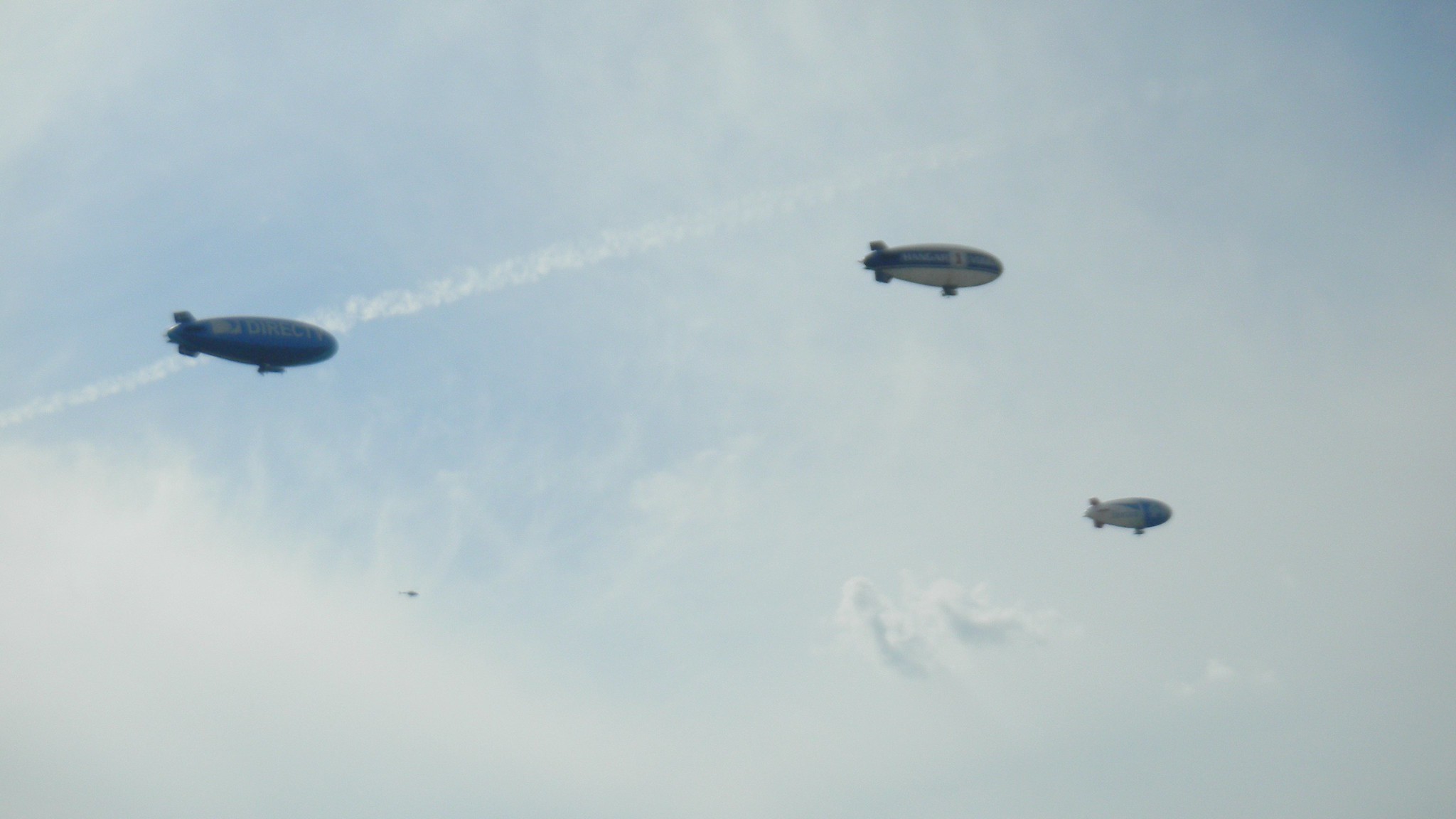This image captures a skyward view of three modern blimps, reminiscent of the Goodyear types, soaring through a light blue sky with scattered puffy white clouds and a few wisps of cloud coverage. From the ground perspective, the blimps are somewhat out of focus due to the distance, making the details and any writing on them hard to discern clearly. Starting from the left, about an inch into the frame, there's a prominent dark blue blimp with some indistinct gold writing, possibly "DIRECTV." In the center-right, slightly further back, there's another blimp featuring a white bottom and blue sides, adorned with some yellow text that is difficult to read. The third blimp, positioned to the far right and farther back, appears blue and white but is mostly just an outline due to its distance, with a noticeable blue front and a white rear. Additionally, a thin smoke trail extends diagonally from the middle left of the image towards the upper right corner. All the blimps are flying in the same direction from left to right, creating a dynamic composition in the serene sky.